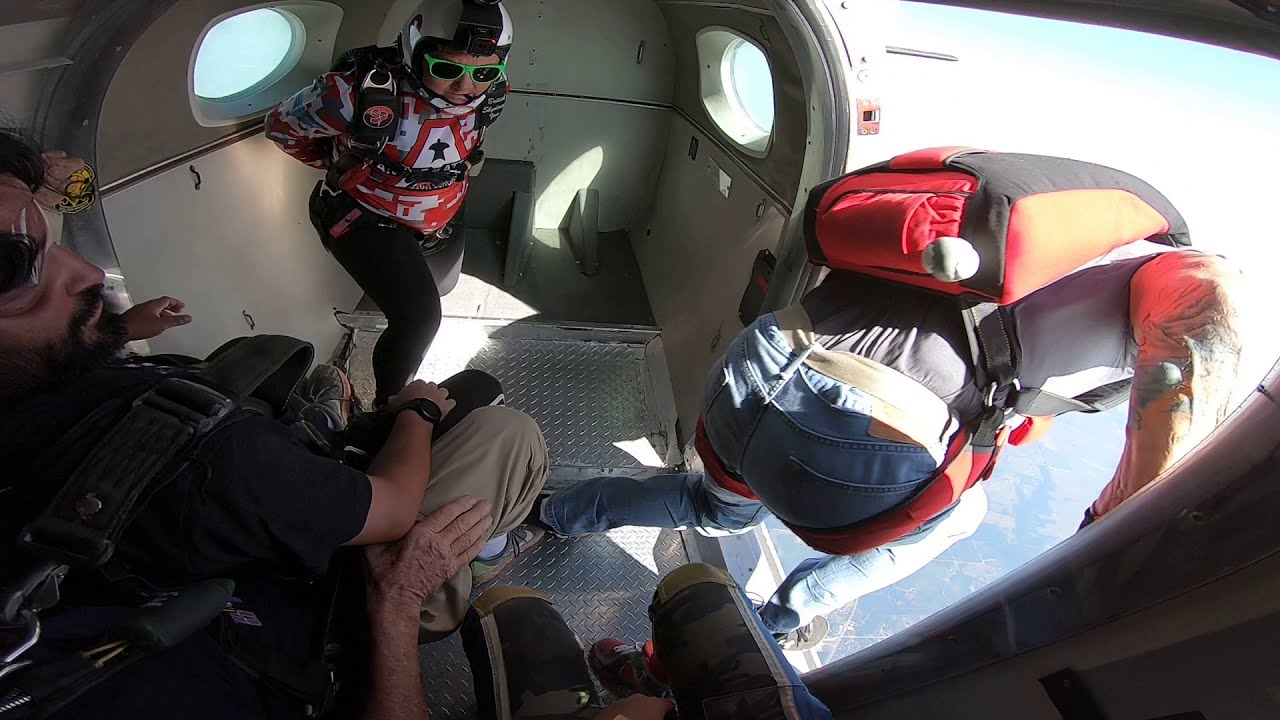The photograph captures an intense moment inside an airplane as four individuals prepare for a skydiving adventure. On the right side, the plane's door is open, revealing a view of the landscape far below. A muscular man in blue jeans and a gray shirt stands poised to jump, his red and black parachute strapped securely to his back. Behind him, a middle-aged woman stands in a white helmet with a mounted camera, green-rimmed sunglasses with black lenses, and a white and red jacket, paired with tight black pants. Seated on the left, a man with a mustache and beard wears a black shirt, tan pants, black wristwatch, and a black parachute, ready to join the excitement. Partially visible in the foreground is another person, whose black camouflage shoes with black and red tennis shoes hint at their readiness. The image vibrates with the anticipation and adrenaline of the imminent jump.